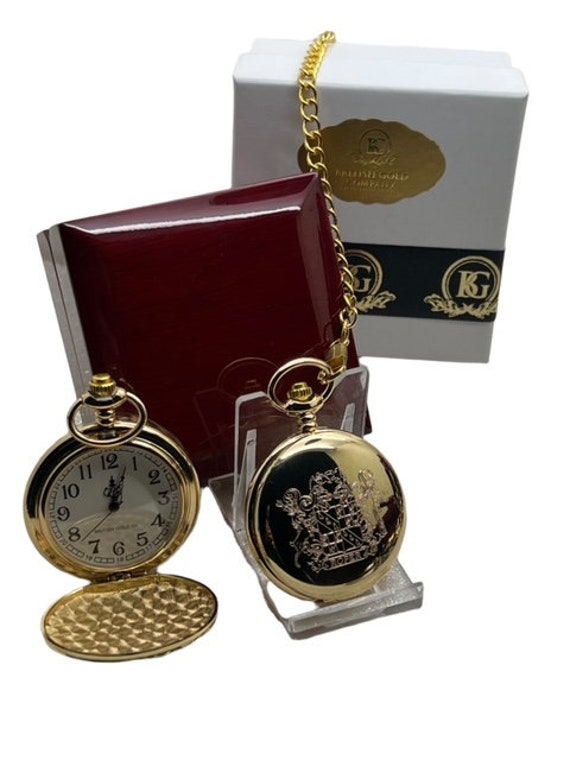The photograph showcases a collection of elegant jewelry, primarily featuring two gold pocket watches. Positioned at the bottom left of the image, one watch is open, revealing an ornate clock face adorned with numbers in a fancy font and decorative clock hands. To its right, another pocket watch is displayed on a small plastic tray stand. The front cover of this closed watch is intricately engraved with a royal coat of arms design. A delicate gold chain extends from this watch, draping over a white box situated in the background. 

This white box, which resembles a jewelry case, features a black ribbon with a gold logo marked "BG" encircled by olive branches. Additionally, the box displays an oval gold sticker bearing the same BG logo. Behind the plastic stand holding the closed watch, a red velvet jewelry casing is visible. The overall composition is devoid of any external background elements, focusing entirely on the luxurious items and their sophisticated presentation.